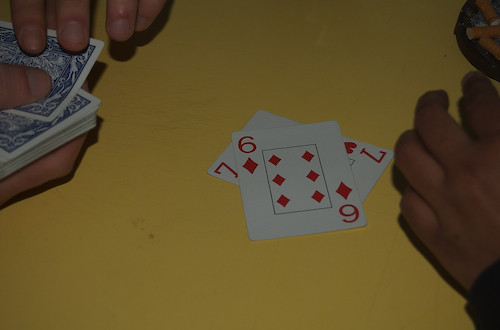In the image above, two individuals are engaged in a game of cards on a vibrant yellow surface that creates a bright and lively background. Lying on the table are two playing cards: the red six of diamonds and the red seven of hearts. The person positioned on the far left of the image holds a deck of cards, suggesting they are the dealer. On the right side, a single hand is visible, dressed in a long-sleeved shirt or jacket, with the wrist prominently shown.

In the upper right corner of the image, there is a partial view of a cartoon character, which appears to depict a female figure, adding a whimsical touch to the scene. The focus on the hands and cards, combined with the vivid yellow background and the playful cartoon, creates a dynamic and engaging visual narrative.